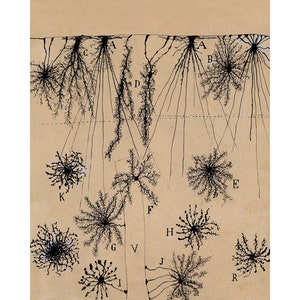This image is of a tan-colored piece of paper that has been scanned, showcasing various intricate designs in black and gray. At the top of the image, approximately an eighth of the way down, there's a horizontal line from which multiple plant-like illustrations hang. These plants vary in appearance: some resemble clusters of twigs or vines without leaves, forming fan-like shapes, while others mimic the form of dandelions gone to seed, with pinwheel-like flowers. The designs bear a static-like quality and seem almost spider-esque in their intricacy. The plants are all labeled with letters ranging from A to R, though no key is provided to explain what these labels signify. The detailed and repetitive nature of these botanical designs creates a compelling and abstract visual ensemble across the tan background.